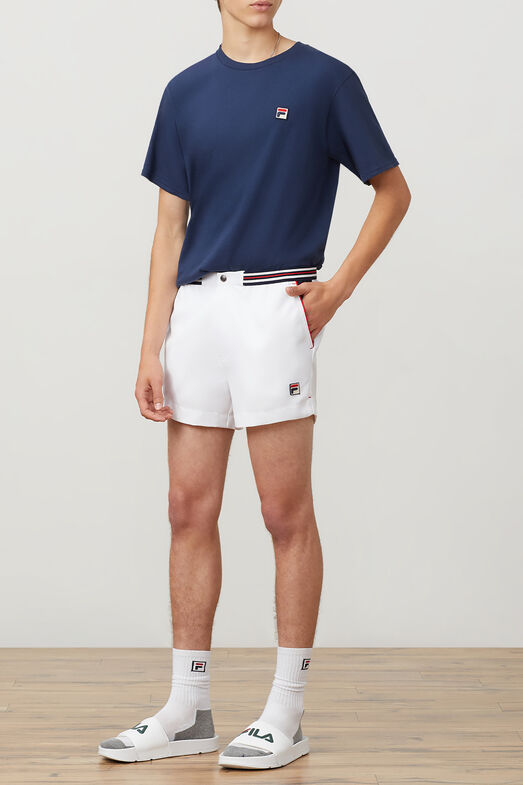The image depicts a young, tall, and fit man modeling FILA brand clothing, standing on a hardwood floor with a white wall behind him. The photograph cuts off just above his lips, revealing only a sliver of his black hair, and he is posed with his left hand in his shorts pocket and his right hand curled by his side. He is wearing a navy blue FILA t-shirt featuring the brand’s red, white, and blue logo on the left breast. His white shorts, which end mid-thigh, have distinctive red and black stripes at the bottom right and a red, white, and blue striped belt. The FILA logo appears again near the bottom of the shorts. Completing his outfit are white FILA socks, noticeable for their gray and red "F" logo, and white FILA slide sandals with gray text on the band. The model's stance has his head turned slightly to the right while his feet are positioned towards the left, highlighting the athletic and stylish nature of the ensemble.